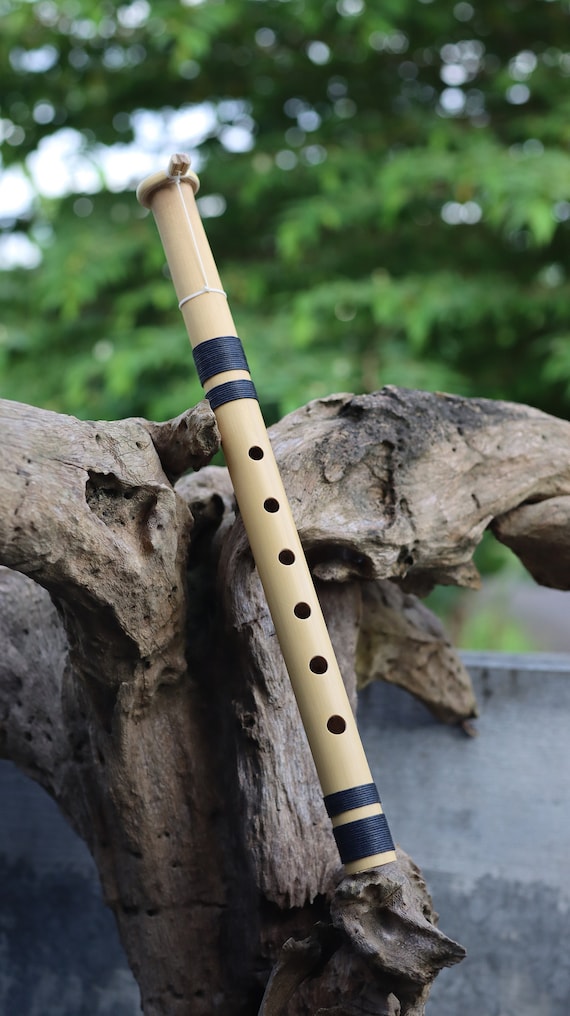The photograph is a tall, portrait-mode image showcasing a handmade flute-type musical instrument positioned diagonally from the bottom right to the top left corner. The flute, resembling a recorder, is crafted from a beige or cream-colored material, possibly a plastic pipe, and features six hand-drilled holes along its length. It is decorated with black tape bands, four in total, with one band at the upper end and another about three-quarters down its length, where the holes end. Additionally, a white string is visible near the top. The flute is set against an old piece of driftwood or petrified wood, which is resting on a concrete surface. The background consists of out-of-focus green trees, indicating that the photograph was taken outdoors during daylight hours. The overall color palette of the image is muted, with browns, greens, and subdued tones of beige and blue.